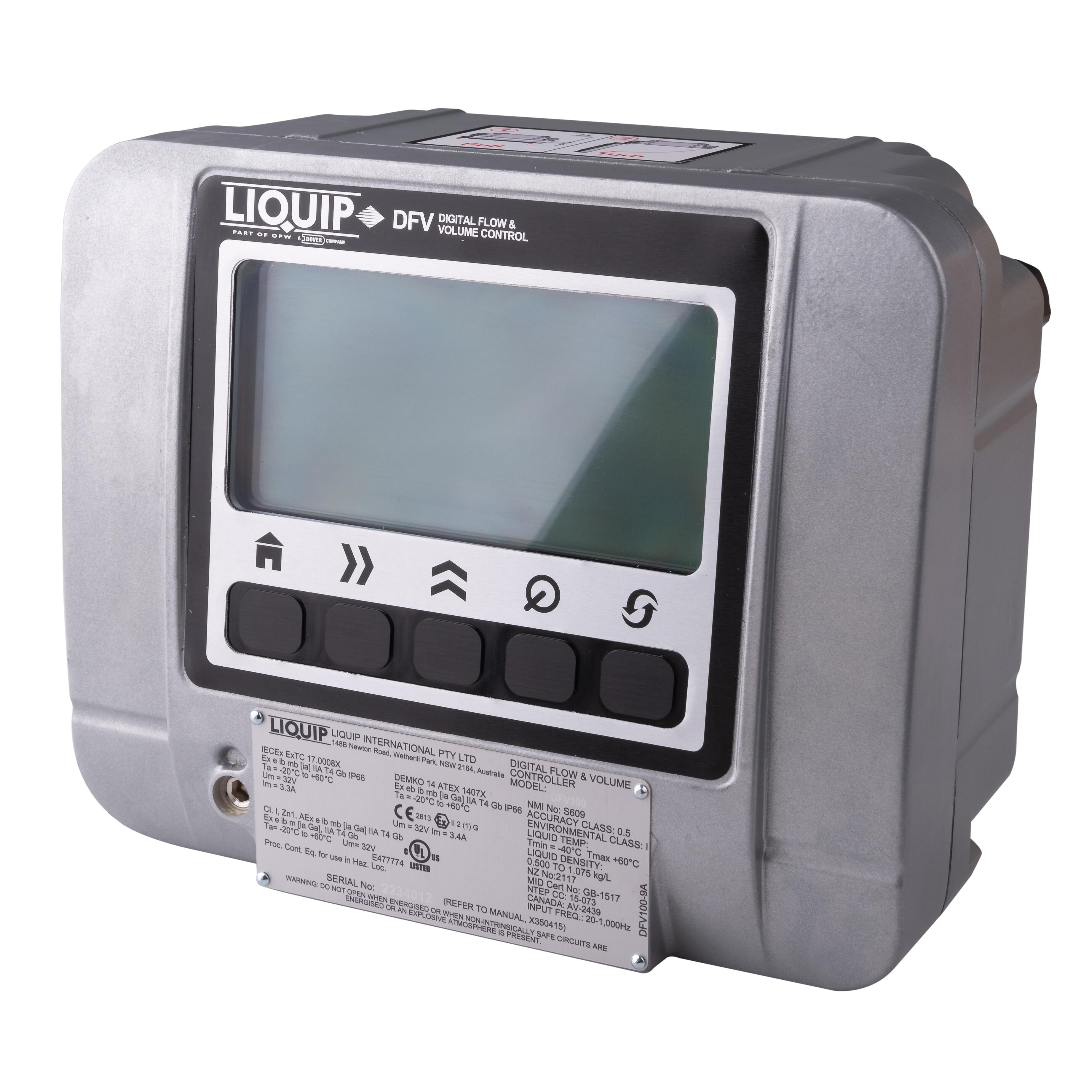The image depicts a large, electronic device with a gray, metallic body and black detailing around the display and controls. At the top of the machine, in white font, it prominently displays the brand "LIQUIP" accompanied by a diamond-like symbol, and the model designation "DFV" followed by the descriptor "digital flow and volume control." The device features an LCD screen that is currently off, situated above a row of five black buttons. Each button has an icon: a house silhouette representing home, two arrows pointing right, two arrows pointing up, a knob set to zero, and a spin-recycle symbol with two rotating arrows. Below these controls is a metallic placard riveted to the device, which reads "LIQUIP International PTY LTD, digital flow and volume controller," followed by the model number and additional specifications. On the left side of this placard, there is a jack opening. The overall appearance and labeling suggest this device is used for precise fluid management.